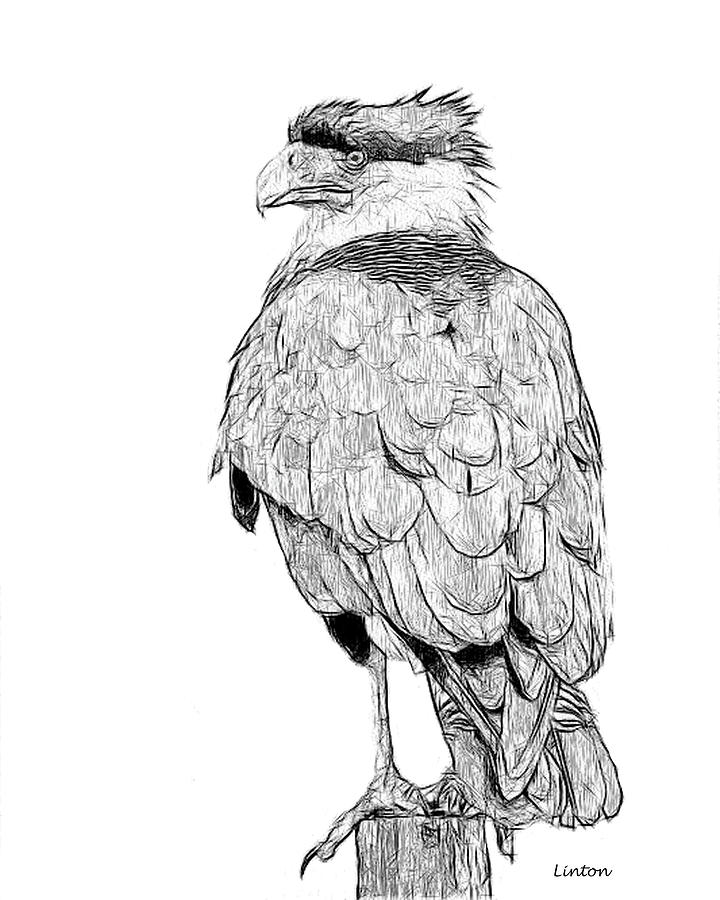This image is a meticulously detailed pencil or charcoal drawing of what appears to be a falcon or eagle, standing on a thick, long wooden post. The bird is captured in a profile shot, looking off to the left, with only the side of its face visible. Its head, characterized by a flat top and prominent beak that points downwards, displays a striking contrast of white around the face and neck, and darker shades on top. Feathers protrude from the back of its head, adding to its lifelike appearance. The bird's wings and tail feature peculiar horizontal stripes, enhancing the depth and texture of the illustration, which employs a crosshatch-heavy style to accentuate its 3D effect. The background remains pure white, allowing the intricacies of the bird to stand out. Notably, the drawing is signed by Linton in the bottom right-hand corner.